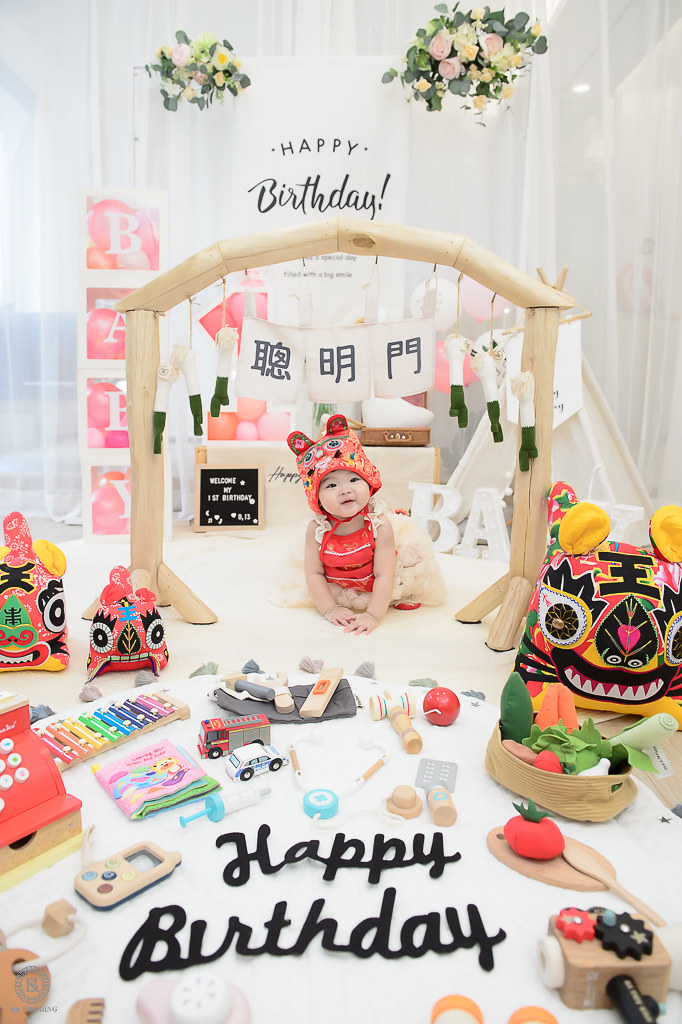In this delightful birthday-themed photo shoot, a cute baby, possibly of Asian descent, takes center stage in a traditional and colorful setting. The baby, wearing an adorable red hat with ears and a red bib over a white outfit, is positioned in a half-crawl on a pristine white floor. The floor features "Happy Birthday" written in black letters at its center, with the same message displayed prominently at the top. Surrounding the baby is an array of toys including a clay tomato, a toy cashier, a pacifier, colorful balls, little cars, musical toys, and more. Chinese characters grace a decorative archway above the baby, adding a touch of cultural significance, possibly indicating the baby's traditional name. The backdrop comprises sheer white curtains adorned with pink decorations, hanging flowers, and plush fabric dragons, creating a festive and vibrant atmosphere much like a meticulously arranged department store photo setup.